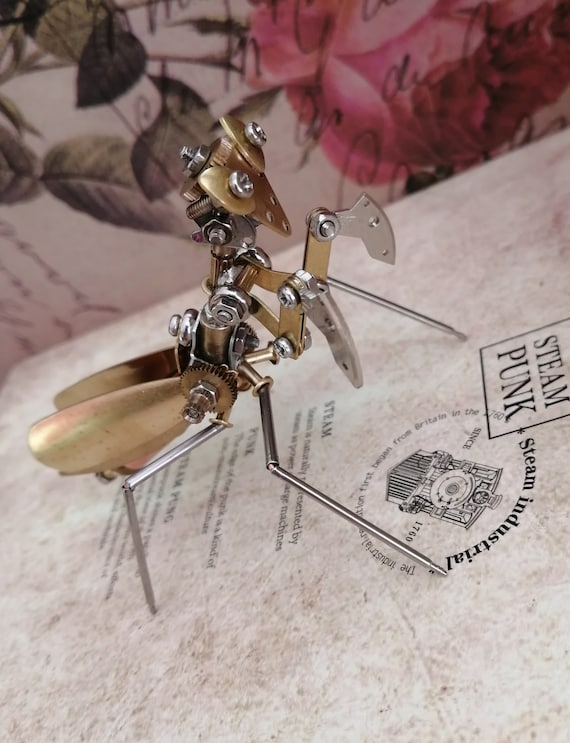This detailed photograph showcases a small mechanical sculpture designed to resemble a praying mantis with a distinctive steampunk aesthetic. Positioned on a slightly dirty white piece of paper that reads "STEAM PUNK" and features a circular emblem with the text "STEAM INDUSTRIES," this intricate sculpture boasts finely crafted details that blend both bronze and silver metallic parts. The text further mentions historical context about industrialization beginning in Britain in the 1760s and includes an image of a train within the emblem. The mantis-like sculpture is assembled from various screws, nuts, bolts, and gears, featuring elongated front legs and shorter back legs made from silver metal. Its arms are composed of curved metal claws and gold-colored components, meticulously held together by screws and bolts. The head is uniquely fashioned from a gold triangular plate with attached gears, complemented by gold plates with screws serving as eyes. The wings are represented by long, gold metal pieces extending from the back. In the background, there's a secondary piece of paper adorned with a pink and white floral pattern, complete with green and brown leaves, contributing an additional layer of visual detail to this captivating steampunk creation.